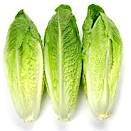The image is a very small, low-resolution photograph depicting three heads of romaine lettuce, arranged vertically side by side against a plain white background. Each head is narrow and oblong, with a white base transitioning into yellowish-green, and then into darker green towards the top. The white veins of the leaves are visible as vertical stripes running up from the base. The lettuce heads are touching each other, with the lettuce in the middle appearing the greenest, especially towards the tip, while the one on the left is slightly smaller. There is no text in the image, no people, and the only colors present are varying shades of white and green. This image appears to be from a shopping catalog or an online retailer's inventory, showing a detailed and structured view of the produce for selection.